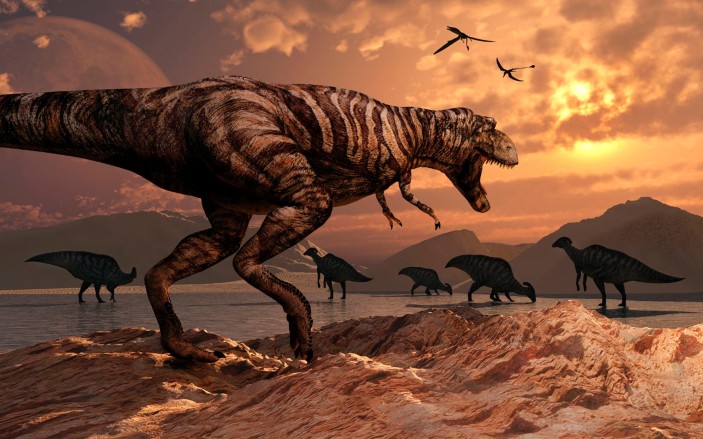In this striking prehistoric scene, a Tyrannosaurus rex stands prominently in the foreground, its mouth agape and head oriented towards the right, with its tail extending out of the frame to the left. The dinosaur's body is adorned with a zebra-like pattern of dark and light brown stripes that run from its small arms to its strong, large back legs. The T. rex stands on a rough, stony terrain that could be a sandy beach under the orangey hues of either a sunset or sunrise. 

In the background, five shadowy figures of dinosaurs, potentially other T. rex, are partially obscured by the dim light. These silhouettes are situated in a shallow body of water, enhancing their mystique. The vast, fantastical sky is filled with dramatic elements, including an ominously large moon occupying a significant portion of the right-hand side, partly veiled by clouds. There are also a couple of pterodactyls soaring high above, adding to the ancient atmosphere. The distant horizon is outlined with low, rugged mountains, further grounding this vivid depiction of the dinosaur era.